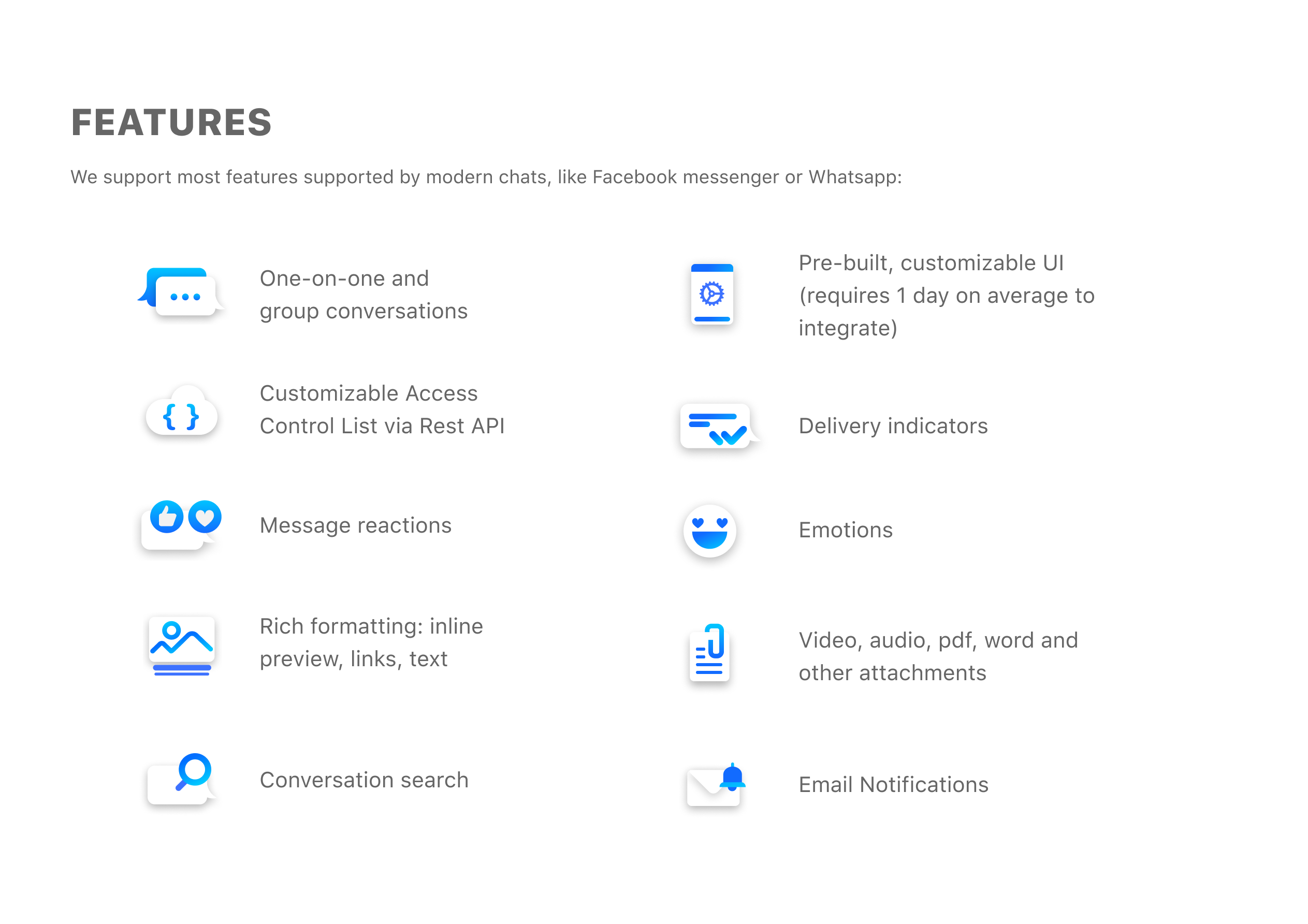The image appears to be a square screenshot from a computer screen, showcasing a detailed list of features offered by a modern chat application. At the very top of the image, there is a prominent heading in large black capital letters reading "FEATURES." Directly below this, the word "FEATURES" repeats in smaller black letters, underlining the theme of the content.

The first feature is highlighted with two speech bubbles: one is blue with a left-facing tail, and the other is white with a right-facing tail containing three blue dots. Accompanying text reads, "One-on-one and group conversations."

Next, there is an icon of a white cloud with blue brackets, alongside text that states, "Customizable access control list via REST API."

Following this, a speech bubble with a blue circle and white thumbs up, paired with another blue circle containing a white heart, signifies "Message reactions."

The subsequent feature is depicted with an image of a white computer screen showing wavy black lines (resembling mountains) and three blue circles, labeled "Rich formatting with inline preview links."

A white box with a blue magnifying glass indicates the capability of "Conversation search."

At the top right of the image, an illustration representing a smartphone with blue bars at the top and bottom, featuring a blue spiky circle with a triangular play button, denotes "Prebuilt customizable UI (User Interface)." The text beneath mentions it takes "one day on average to integrate."

A right-pointing speech bubble with three blue bars of varying lengths and a blue check mark represents "Delivery indicators."

A white circle displaying a face with a blue mouth and heart-shaped eyes symbolizes "Emojis."

An emblem resembling a document with short and long blue lines, partly covered by a blue paperclip, highlights the capability to share "Video, audio, PDF, Word, and other attachments."

Lastly, an icon of a white envelope with a blue bell at the top right corner signifies "Email notifications."

Overall, the image describes an array of advanced chat features typically found in modern messaging apps similar to WhatsApp or Facebook Messenger.